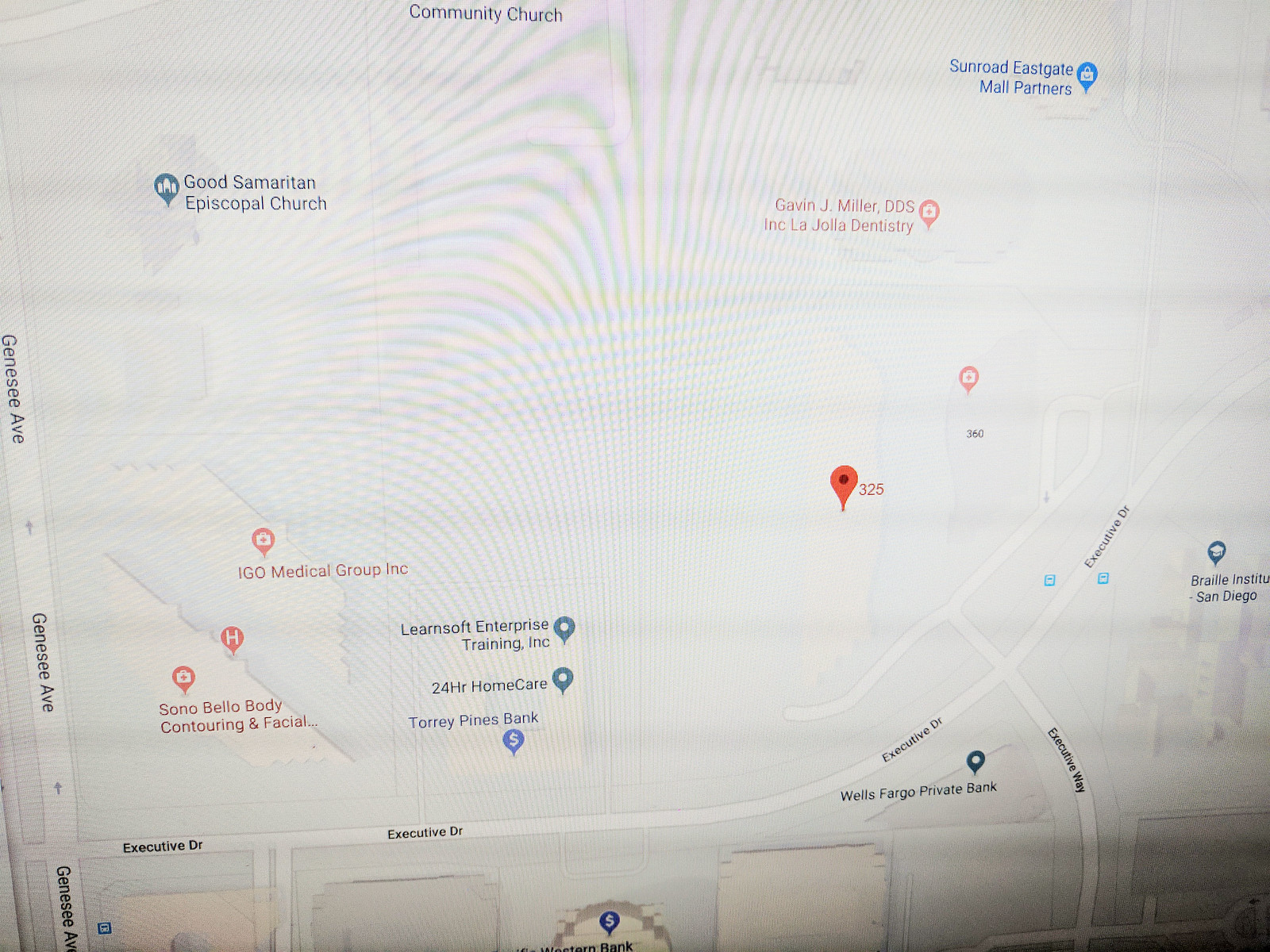This image displays a detailed map on a computer screen. Prominently featured at the top is the "Community Church." On the right side of the map, below "Sun Road Eastgate Meal Partners," there’s "Calvin J. Miller DDS Inc. La Jolla Dentistry." To the left, "Good Samaritan Episcopal Church" is highlighted. The map shows "Genesee Avenue," which runs down to "Executive Drive," intersecting with "Executive Way."

Locations on the map include notable landmarks such as "IGO Medical Group Incorporated" and a hospital marker. Other institutions identified are "Son of Bello Body Contouring and Facial," "Team Soft Enterprise Training Incorporated," "24 Hour Home Care," and "Torrey Pines Bank." 

A noticeable pen marker is placed at "325" near the "Braille Institute San Diego." The map also shows "Wells Fargo Private Bank," situated at the bottom center of the image. While another bank is depicted at the very bottom center of the photograph, its specific name remains unreadable.